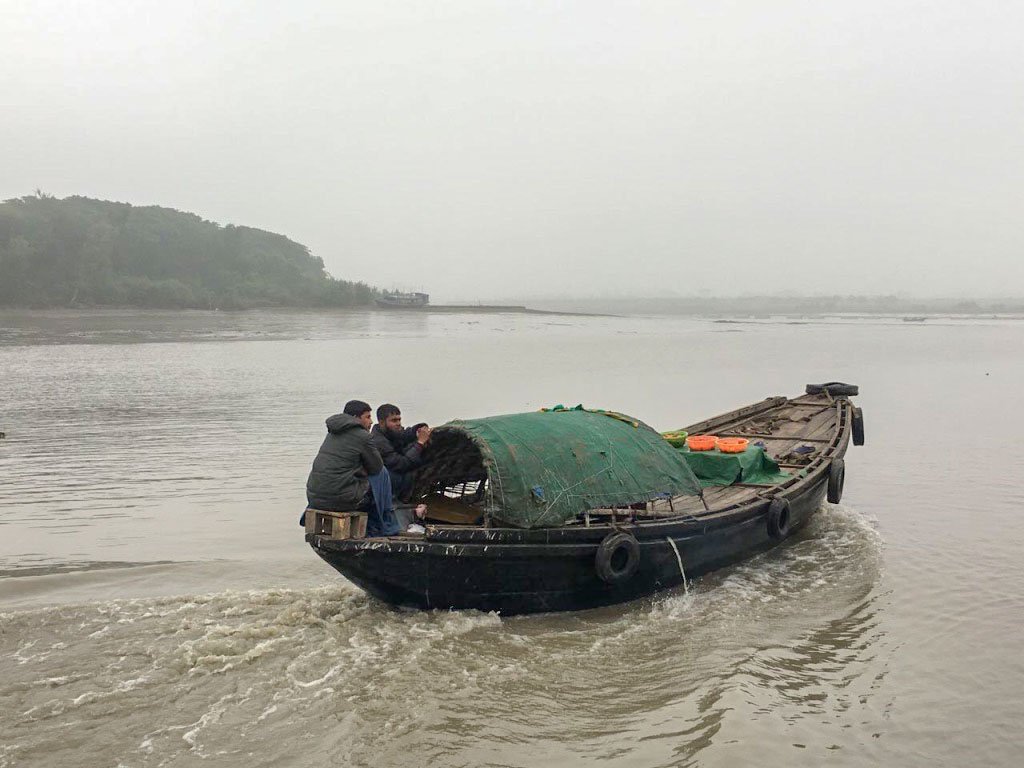In this evocative image, two fishermen of Indian descent navigate the murky waters of the Bay of Bengal in a weathered, derelict boat. Dressed in practical black puffer jackets and denim pants, they brace against the elements under a small green awning tarp that provides scant shelter. The boat's age is evident from its condition, notably marked by a couple of tires acting as makeshift bumpers. Centrally placed on the boat is a green table cluttered with orange and green bowls, presumably holding fishing supplies. The atmosphere is dominated by a gray, overcast sky that mirrors the slate-colored waters below. In the distant left, a hint of green landmass—possibly an island—breaks the monotony of the horizon. Despite the bleak and murky setting, the image captures a poignant moment of these fishermen embarking on their daily labor in what appears to be their own personal fishing vessel.